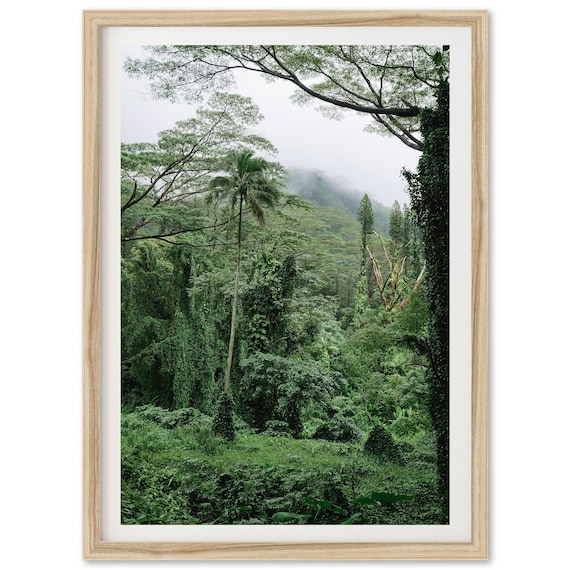"Framed in a light brown wooden frame with a white mat, this vertically oriented color photograph captures the lush, untamed beauty of a tropical jungle or rainforest. Dominating the scene slightly to the left of center is a tall palm tree, its fronds reaching skyward amidst a dense tapestry of green foliage and moss. The vibrant hues of dark and light greens are interspersed with subtle blue undertones, while a layer of fog rolls in over distant hills, adding a sense of mystery. The overcast, white sky casts a muted light over the verdant landscape, emphasizing the wild and overgrown nature of this tropical setting."